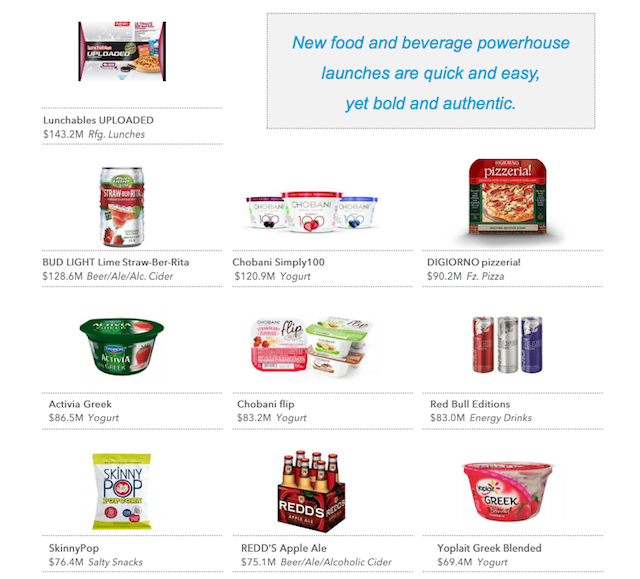In this image, a variety of food and beverage items are prominently displayed, totaling ten distinct products. Each item is accompanied by its respective price. The showcased products include:

1. Lunchables - Priced at $1.43 each, these are convenient, pre-packaged meal kits.
2. Bud Light Lime Strawberry Tea - Each can is priced at $1.28, offering a refreshing blend of flavors.
3. Chobani Simply 100 Yogurt - Each cup costs $1.20, known for being a low-calorie yogurt option.
4. DiGiorno Pizzeria Pizza - Each box is priced at $9.02, featuring gourmet-style frozen pizza.
5. Red Bull Editions - These energy drinks are remarkably priced at $3.00 each.
6. Yoplait Greek Blended Yogurt - Each cup is tagged at $6.94, known for its smooth texture and rich flavor.
7. Red's Apple Ale - Valued at $5.10 per bottle, this is a crisp apple-flavored beer.
8. Skinny Pop Popcorn - A bag costs $6.40, acclaimed for being a healthier snacking option.
9. Activia Greek Yogurt - Each container is priced at $6.50, noted for its probiotic benefits.
10. Chobani Flip Yogurt - Each unit is valued at $3.20, combining creamy Greek yogurt with tasty toppings.

The composition of this image underscores a mix of everyday essentials and specialty food items, each clearly labeled with their price, providing a comprehensive overview of the displayed products.